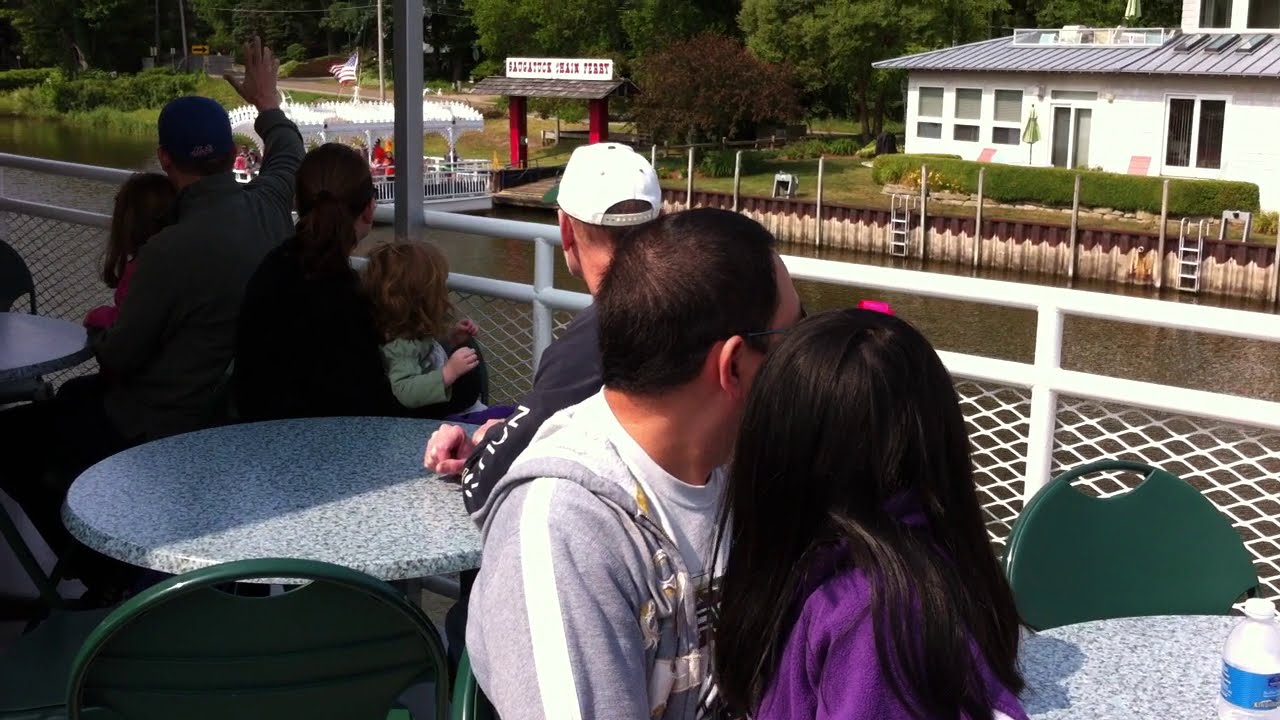In this detailed picture, a group of seven people are seated on a boat that is gliding along a brown waterway, possibly a canal or river. They are at three circular tables with green chairs. The scene captures a relaxed, social atmosphere. Prominently in the foreground are two people with their backs to the camera. One is a woman with black hair wearing a purple sweater, and the other is a man with black hair and glasses, donning a gray hoodie with a white stripe along the arm and a white T-shirt underneath.

Next to this couple sits a man with a white baseball cap, facing the water. Further along, a family of four is gathered at another table with a mix of children and adults—one child with short hair, possibly blonde or brunette, and a woman with her hair in a ponytail who is dressed in a dark top. A man with a blue hat, also wearing a dark, long-sleeved top, is waving towards a boat in the background. This background boat, which is a white pontoon-style vessel with a flat surface and railings, is at a 45-degree angle relative to the boat they're on. 

The backdrop also includes a white building with multiple windows and a sliding glass door, nestled among trees and shrubbery. There’s a road and more foliage visible further in the background. The image also reveals some smaller details such as a water bottle on one of the tables, enhancing the everyday, spontaneous feel of the moment captured in this photograph.